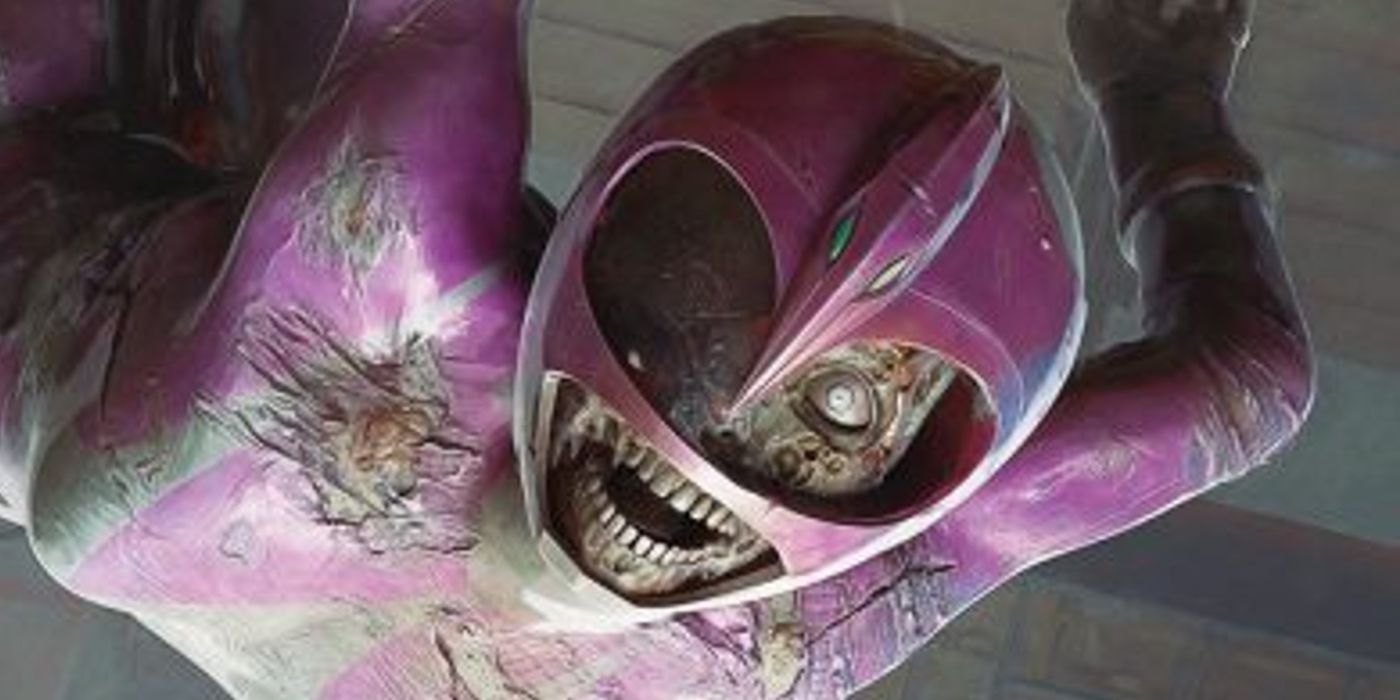The image features a terrifying close-up of a nightmarish creature reminiscent of a Power Ranger. The creature is only visible from the chest up, clad in partially distressed armor that is primarily a pinkish-purple hue accented with silver stripes. The helmet, of the same purple color, features an extruded top piece resembling a reptilian form, tapering to a sharp point and adorned with blue accents and a red and white diamond shape. The skeletal face inside the helmet has a partially visible, lifeless eyeball and a gaping mouth with a full set of teeth, giving it a haunting appearance. The armor appears battle-worn, hinting at prior combat. Background elements are a wooden ceiling and wall, enhancing the unsettling atmosphere as though the creature is lunging toward the camera.